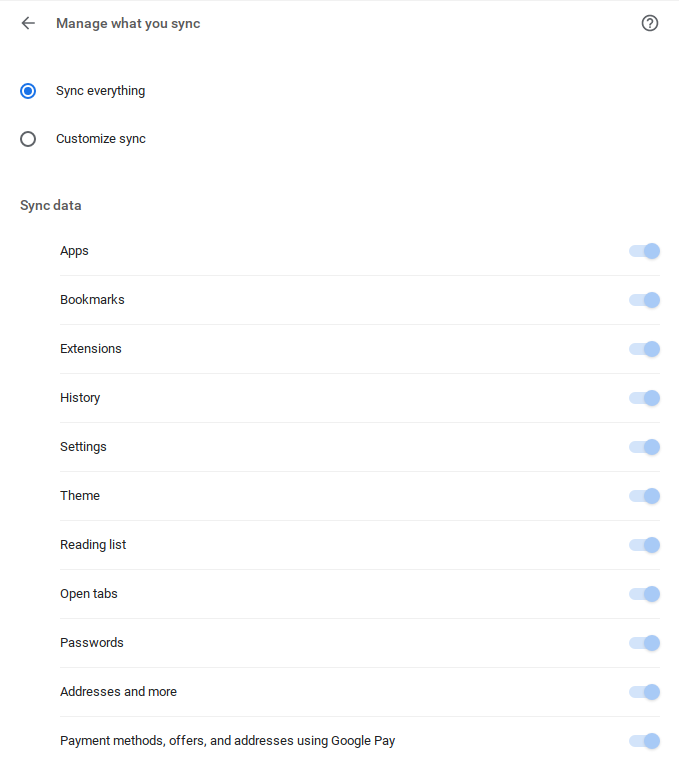The image is a detailed screenshot of the "Manage What You Sync" page within a Google account settings interface. At the top of the interface, the page title "Manage What You Sync" is prominently displayed. Below the title, two radio button options are presented: "Sync Everything," which is currently selected, and "Customize Sync."

Underneath these options, there is a "Sync Data" section, featuring a comprehensive list of items with corresponding toggle switches. Each item is currently toggled on and includes: Apps, Bookmarks, Extensions, History, Settings, Theme, Reading List, Open Tabs, Passwords, Addresses and more, Payment Methods, Offers, and Addresses using Google Play.

To the left of the title, there is a back arrow for navigation, while on the right side, a small question mark icon is visible, likely designed for accessing help or additional information. The design of the page is clean and minimalistic, characterized by a white background and black and blue text, aligning with Google's typical aesthetic for its settings pages. The overall layout is straightforward and user-friendly, ensuring ease of navigation and clarity in managing sync settings.